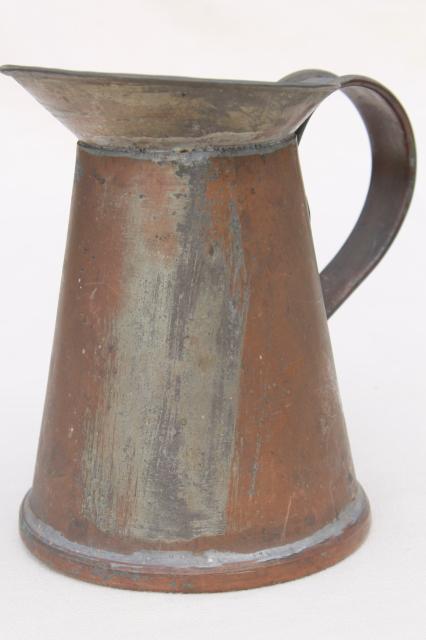The image is a painting, a detailed still life showcasing an ancient, pewter pitcher set against an off-white background. The pitcher, with its cylindrical body and curved handle positioned on the right-hand side, exhibits signs of significant age and rust, rendering it a dull, brown-gray hue. The light reflecting off its surface creates subtle gleams that highlight its discolored, uneven texture. The top of the pitcher features a wide pouring spout, slightly lighter in color yet merging into the darker tones along the rim. Below the body, a scratched area reveals hints of the original pewter beneath the rust. A gray band wraps around the bottom of the pitcher, growing darker at the base. Close inspection reveals a small pinhole two-thirds up from the bottom and weld marks where the spout has been attached. This visual narrative hints at the pitcher’s long history and utilitarian past, evoking a sense of antiquity.